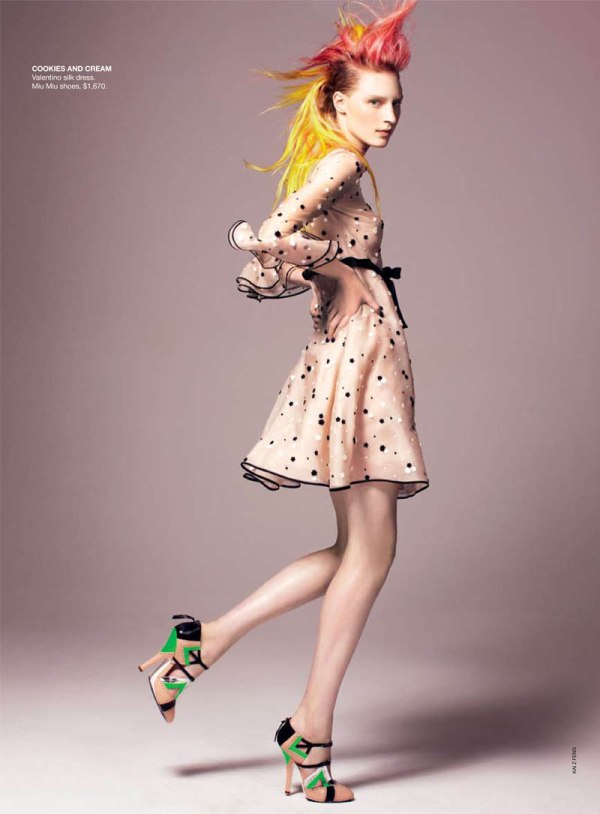The image depicts a tall, very thin, and attractive fashion model in a photo that resembles a full-page magazine advertisement. She stands against a beige background with text in the top left corner that reads "Cookies and Cream," possibly the name or style of the dress she is promoting. The dress is a short, light-colored garment adorned with black and white polka dots and has a black rim around it. A black belt cinches her waist. 

Her hair is styled in an edgy faux hawk, combining shades of vibrant pink and yellow, with pink dominating the top and yellow cascading down her back. She has a cute face and is posed playfully, standing on one foot while the other is kicked back behind her. Her shoes are high heels with black straps that lace around her ankles and feature green and tan accents. Her long legs and arms add to her striking, elegant appearance. Additional small text underneath the main branding mentions "silk dress" and lists a price of $1,600.